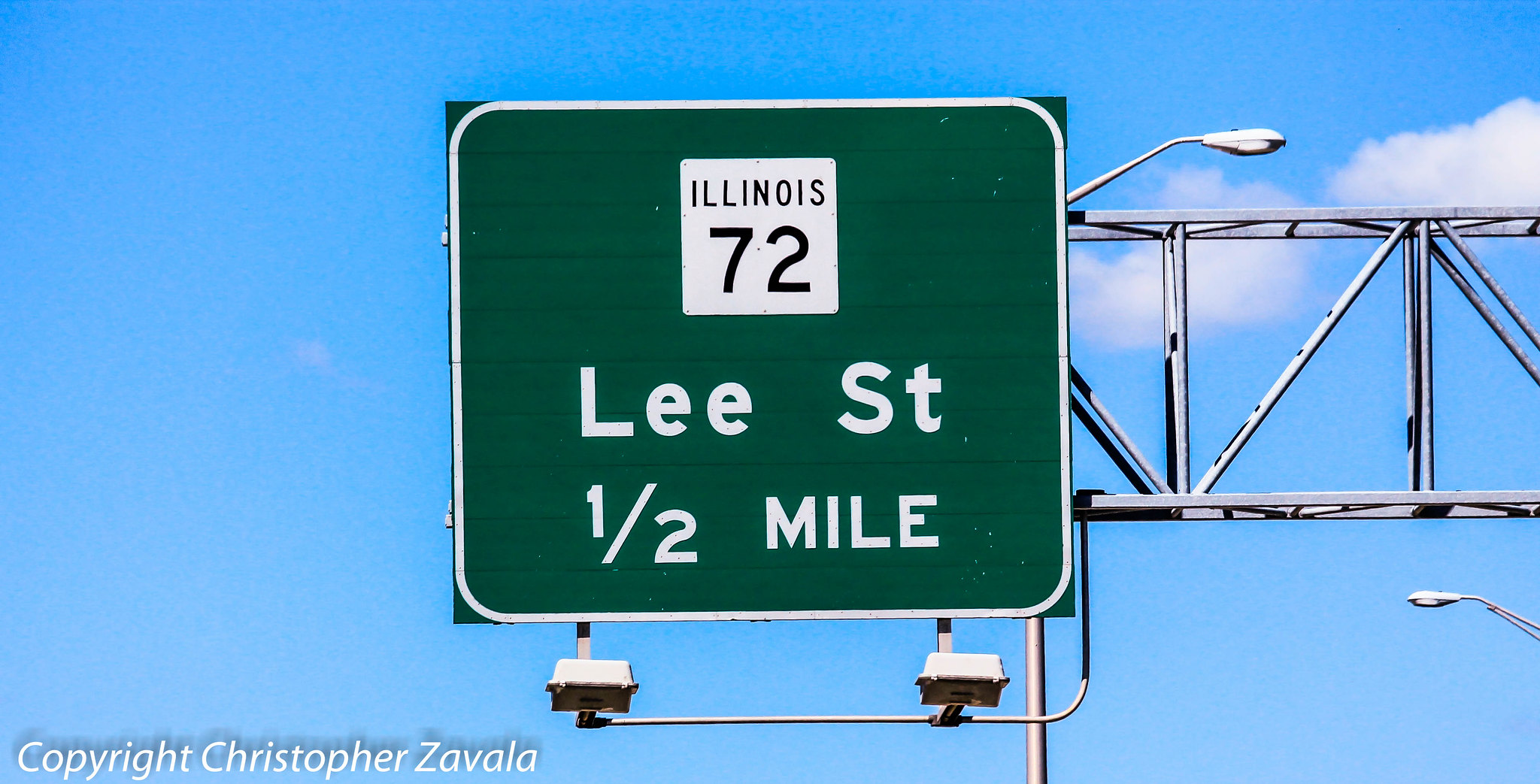The image depicts an outdoor highway sign set against a blue sky with a few clouds on the upper right side. The green rectangular sign, which has a thin white border with rounded corners, takes center stage of the photo. In the middle of the sign is a white square featuring the black text "Illinois 72." Below this white square, the sign displays "Lee Street" in white text, followed by "Half Mile," also in white. Supporting the sign, there are metal pieces visible beneath it, alongside a larger metal structure and streetlights situated to the right. In the bottom left corner, the image bears the copyright notice "Christopher Zavala." The overall aesthetic of the image is pristine, almost as if digitally enhanced, making the highway sign's details and the sky's vibrant hues stand out sharply.